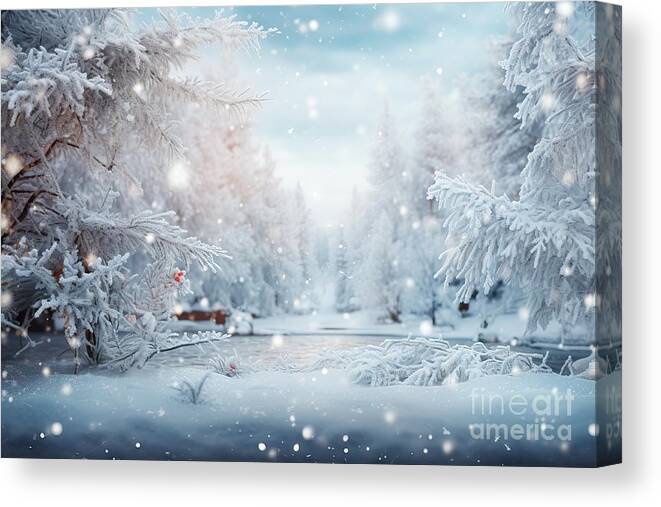The image is of a three-dimensional rectangular canvas painting tilted slightly to the left, set against a white background. The artwork depicts a serene winter scene, featuring conifer trees heavily laden with snow and a partially frozen dark gray lake at the center. The landscape is entirely blanketed in snow, with additional trees in the background that appear white and gray, creating a monochromatic palette. The sky at the top has a rich yet slightly dulled teal hue, with white circular snowflakes gently falling across the scene.

In the bottom right corner of the canvas, there is text that reads "fine art america." The word "fine" is in a larger, thin font, while "art" and "america" are bolded but in smaller font sizes, with all letters in lowercase. The letters are light gray, adding subtlety to the design.

Overall, the digital painting exudes a tranquil, wintry atmosphere, accentuated by details such as reddish flowers scattered among the snow-laden branches on the left and more tall, snow-covered trees to the right.